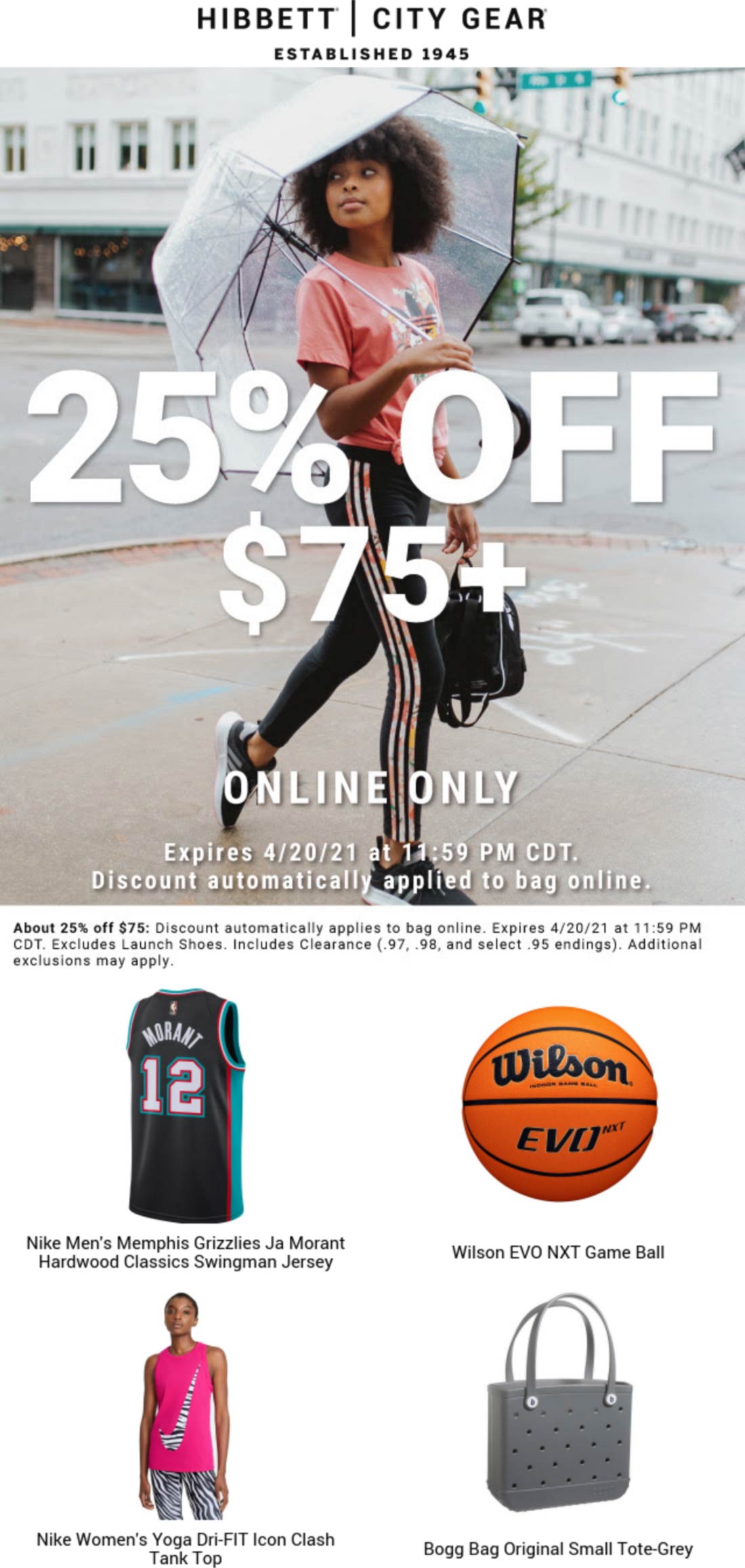Screenshot of Hibbett City Gear website, established in 1945. It features a young woman wearing an orange shirt and black leggings with three stripes along the sides, possibly Adidas, walking on a downtown sidewalk. Parked cars are visible on the street. The woman carries a clear umbrella. Text on the image reads: "25% off $75+ Online only. Expires 4-20-21 at 11:59 p.m. CST. Discount automatically applied to cart online." Additionally, the screenshot showcases four sections: a jersey with "Bryant" on it, a Wilson EVO basketball, a woman in a pink zebra-patterned Nike shirt, and a black tote bag.